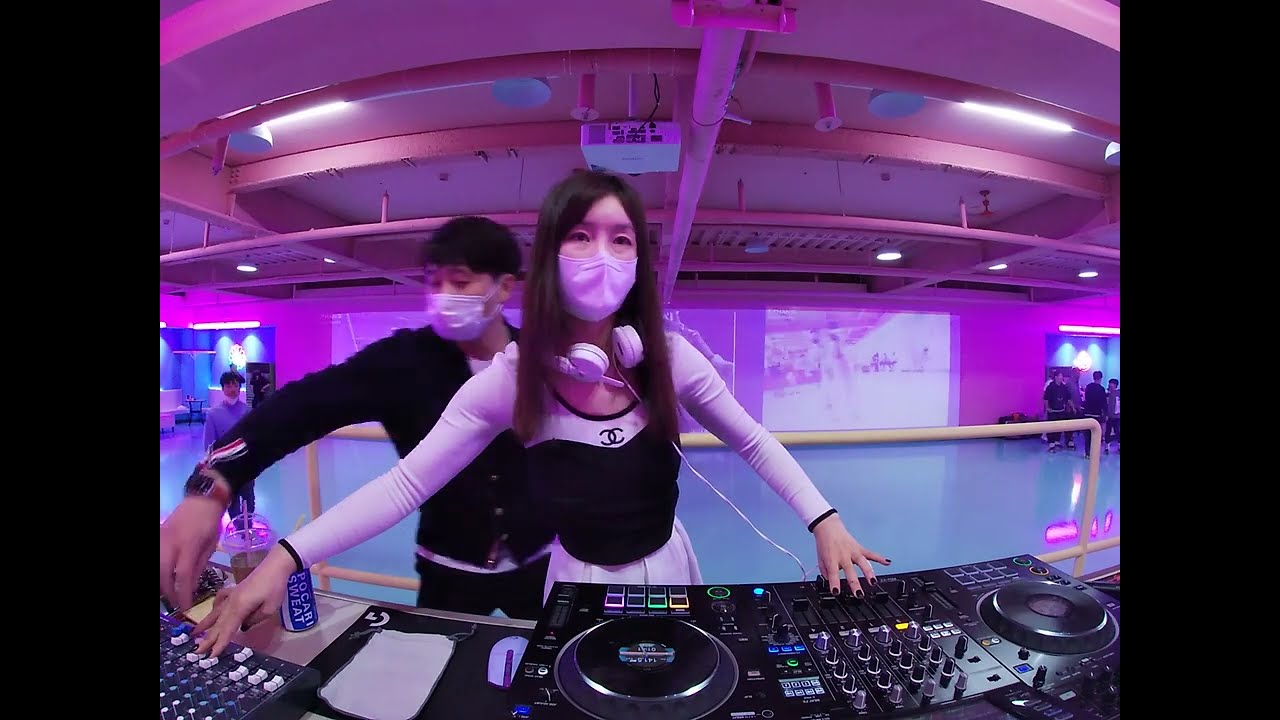The image depicts a vibrant club scene with prominent pink decor. At the center, a young Asian woman, dressed in a stylish Chanel-inspired long-sleeved pink and black shirt with a matching pink skirt, stands engaged in a DJ session. She sports a pink mask and pink headphones draped around her neck, exuding a trendy, coordinated look. In front of her is an elaborate DJ setup, complete with turntables, various buttons, and analog knobs. 

Adjacent to her is a young man with short brown hair wearing a black jacket and black pants, also masked. They appear focused on managing the DJ equipment together. The room features striking pink walls and a pink ceiling, with numerous pink metal pipes running across it, creating a whimsical ambiance. The glossy blue floor suggests an area meant for dancing, and there are multiple people visible in the background and the far-right corner, indicating a lively atmosphere.

Vertical black bars frame the left and right sides of the image, enhancing the club's intimate and energetic vibe. A white handrail behind the DJs serves as a barrier, separating the DJ area from the entrance where more guests are likely walking in.